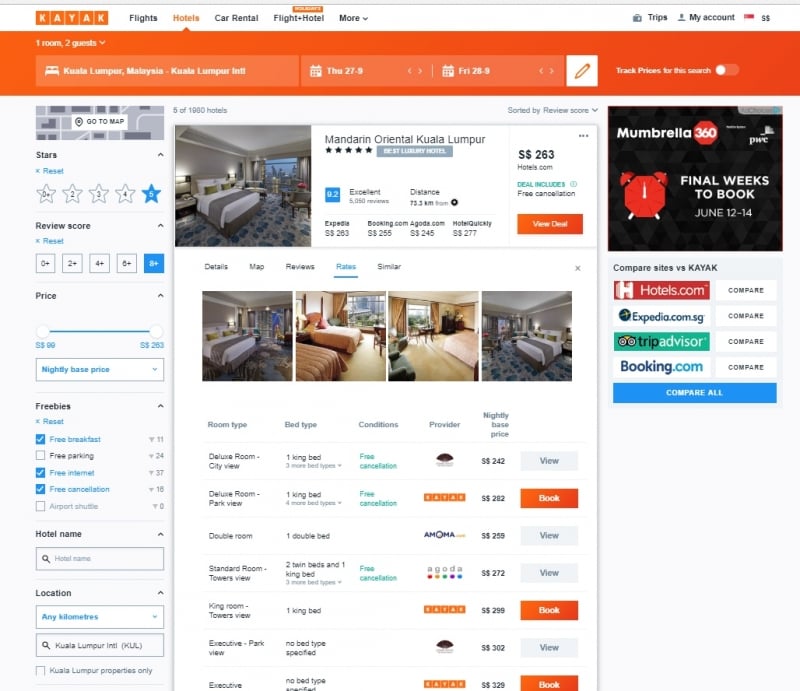Screenshot of a Kayak homepage featuring hotel listings. The user interface includes a left pane with various filters for refining search results. At the top, an orange navigation bar displays the prominent Kayak logo. To the right, advertisements for Hotels.com, TripAdvisor, Expedia, and Booking.com appear, promoting a "Compare All" feature. A light blue bar is present behind these ads, contributing to the webpage's overall design.